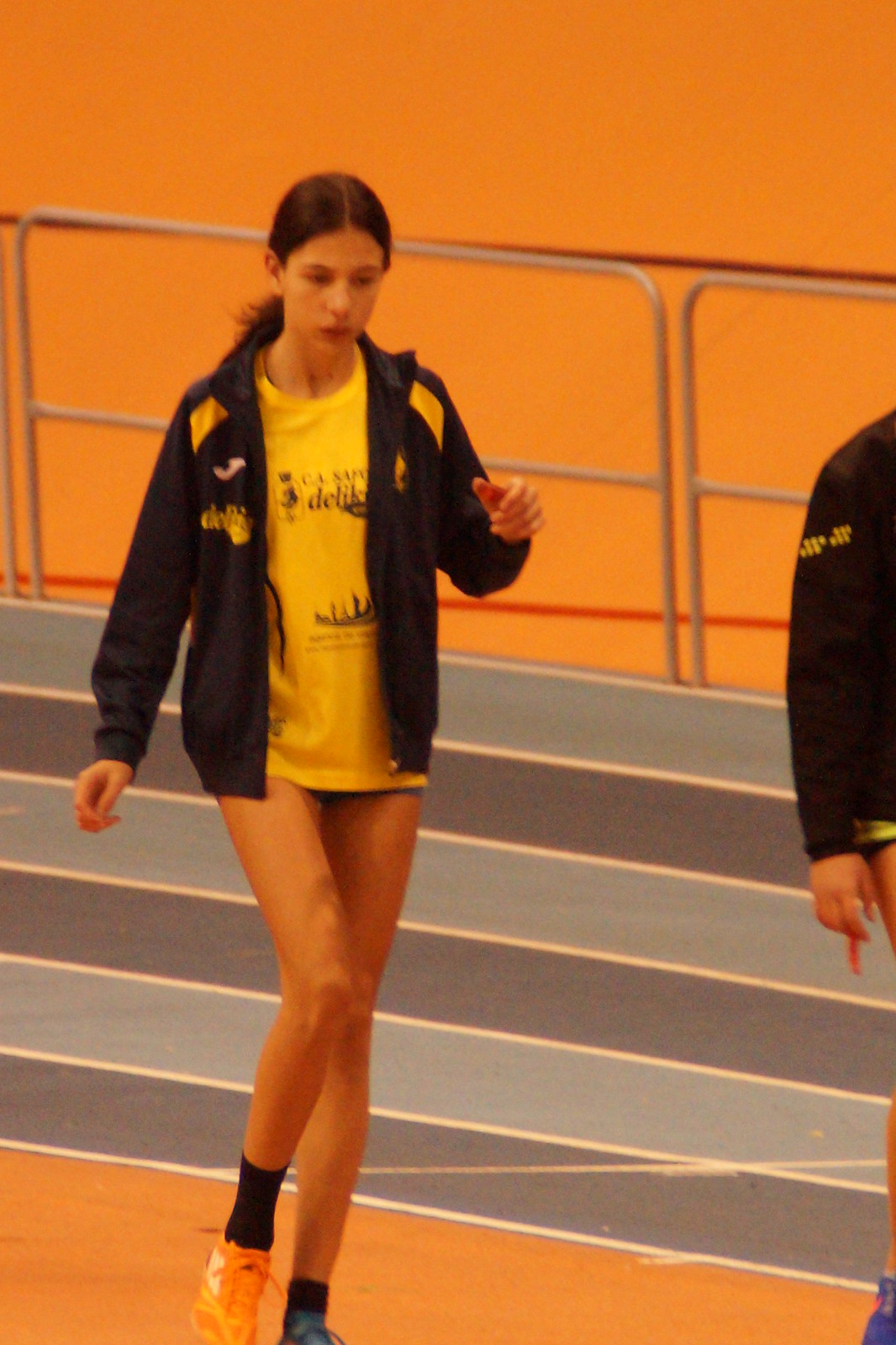This is an image of a young girl with brown hair pulled into a low ponytail, wearing a distinct outfit on an indoor track field. The visually striking track features alternating light blue and dark blue lanes, separated by a metal fence from the bright orange background. The girl is positioned to the left side of the photo and appears to be walking along the area beside the lanes, not on them.

She sports a black jacket with yellow detailing on the shoulders, a yellow shirt with an image of a person rowing a boat, and very short shorts which are mostly obscured by her shirt. Her footwear consists of mismatched sneakers—one orange and one blue, paired with black socks. 

Notably, there's another person in the background, partially visible, seemingly dressed in similar attire and walking in the same direction. The photo itself is slightly out of focus, adding a sense of dynamic movement to the scene.